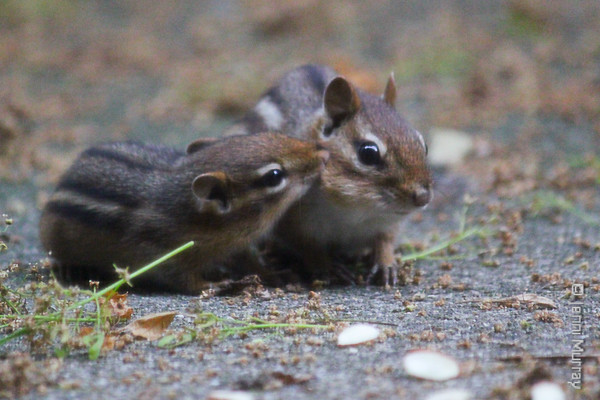In this horizontal nature photo, two dark brown squirrels with black and white streaks lie on a gray, dirt-covered ground scattered with stones, leaves, and green stems. The squirrel on the right is cautiously observing the lower right of the image with a claw touching the ground. The squirrel to the left appears affectionate, pressing its nose into the cheek of the right squirrel as if kissing or comforting it. Both squirrels have dark black eyes, and the right squirrel also has white on its chest and along its back. The background fades into a blurred mix of brown and green, further emphasizing the natural setting. A photo credit to "Jen Murray" is vertically inscribed on the bottom right.